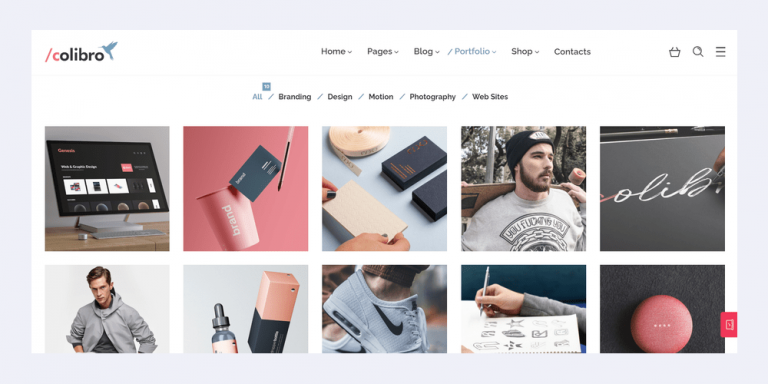Screenshot of the Calibro website, showcasing the Portfolio section. The logo, situated in the top-left corner, features "C-O-L-I-B-R-O" in stylish lettering, complemented by a whimsical hummingbird in flight towards the right. The 'C' is uniquely highlighted in a light red hue, accompanied by a red backslash before it, adding a distinct touch to the branding.

The top navigation bar includes tabs for Home, Pages, Blog, Portfolio, Shop, and Contacts, with the Portfolio tab currently selected and highlighted in blue. Subcategories under the Portfolio tab—All, Branding, Design, Motion, Photography, and Websites—are displayed, with 'All' being the active selection, also highlighted in blue.

The main content area exhibits a variety of visually compelling images, likely showcasing the artistic work and product photography featured on the site. The images include artistic arrangements of products and models donning t-shirts, suggesting that the website may focus on photography and product advertising.